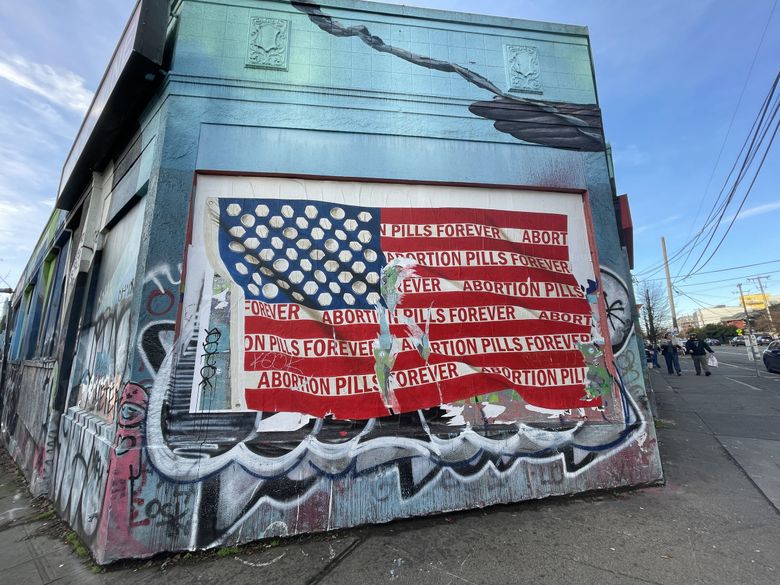The image showcases a concrete building adorned with a mural mimicking the American flag, complete with red and white stripes and a blue field with white dots. The white stripes feature the repeated red text "Abortion Pills Forever." Surrounding the mural is an assortment of graffiti. The building appears somewhat weathered, with a boarded-up window at one corner, and is flanked by sidewalks scattered with dirt. People clad in jackets and pants walk along these sidewalks, with one individual carrying a white bag. The scene includes several buildings in white, tan, and brick hues to the right. Above, electrical wires and a telephone pole cut across a backdrop of blue sky with white clouds, suggesting the time might be early evening.